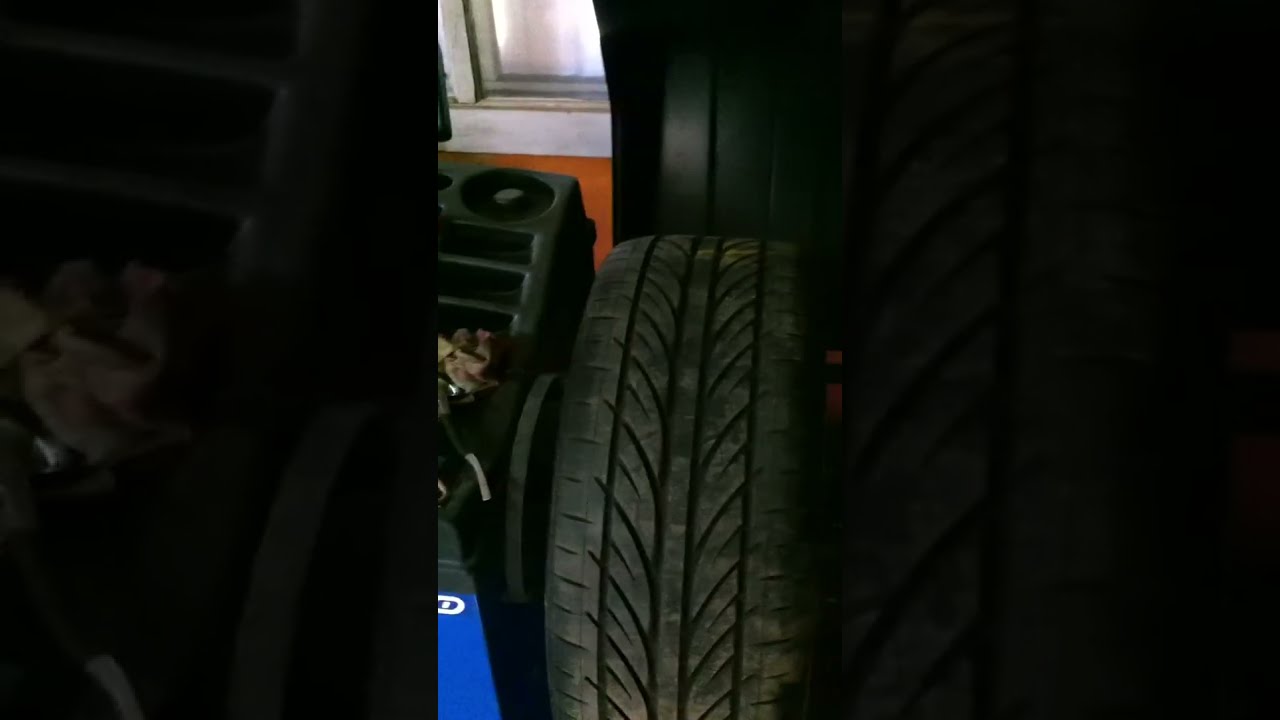The image is a horizontally aligned rectangle with thick black borders on either side, focusing centrally on a somewhat blurry, close-up shot of a large tire, possibly unattached and with visible treads along the top. The background reveals a cluttered workshop setting, featuring an orange-painted wall transitioning into a white section with a dirty window at the top left, stained with what appears to be oil or grease. Below the window, there's a black tray-like equipment with a circular cutout and several built-in slots, suggesting it might be a tool carrier or part of a tire balancing machine typical in automotive shops. The dark surroundings and indistinct details hint that the image might be a screenshot from a video.